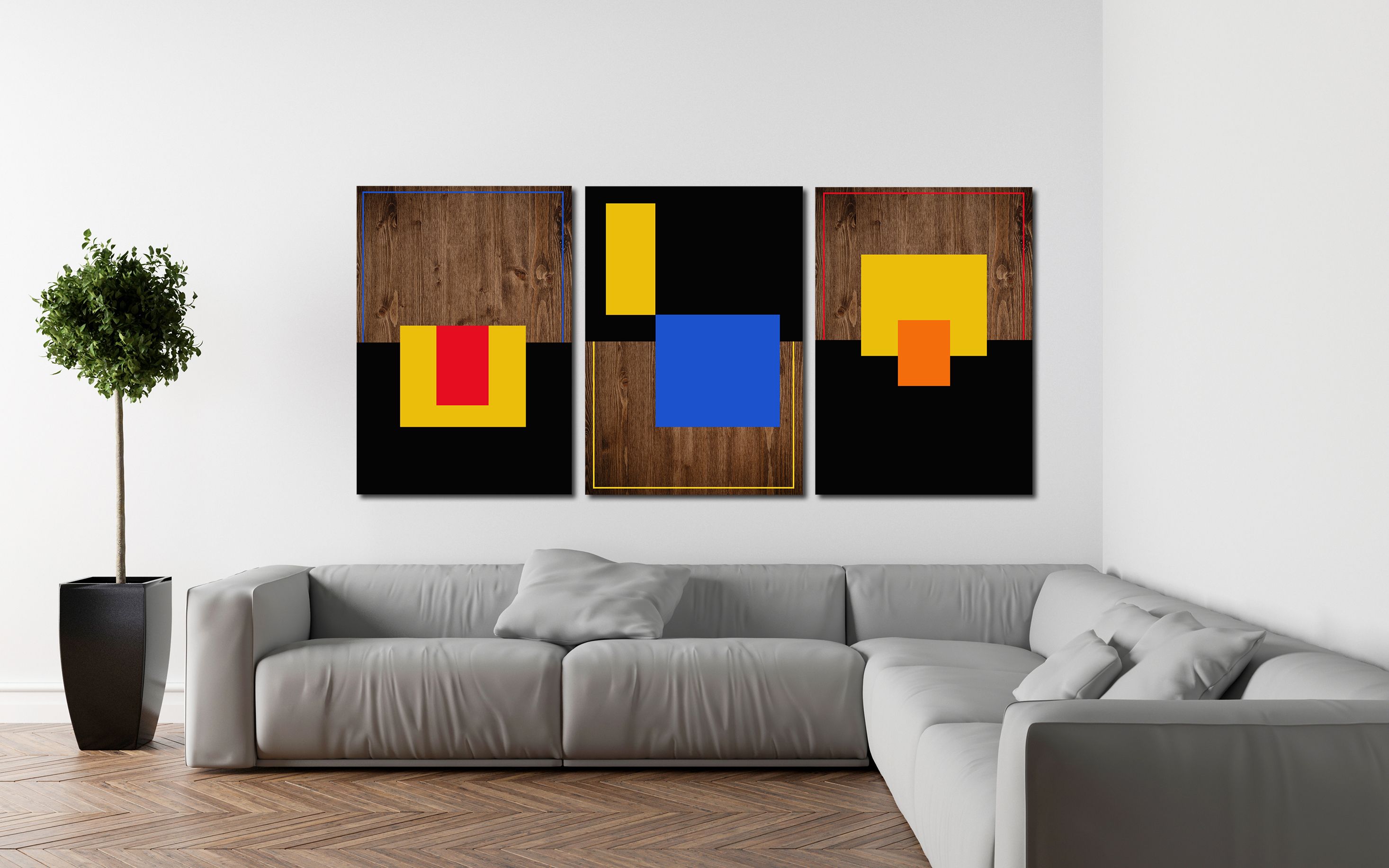The image depicts a meticulously staged product photograph of a modern, minimalist corner room. The main focus of the photograph are three abstract art posters prominently displayed on stark white walls. These posters share a geometric theme, each featuring a base of large brown squares adorned with vibrant blue, yellow, orange, and red shapes, creating a cohesive and colorful visual ensemble. Anchoring the room is a spacious, deep corner couch with plush, grey pillows scattered across its seats, providing ample seating for about eight people. The floor boasts a chic chevron-patterned wooden design, adding texture and warmth. To the left of the couch, a sleek, tall planter in a black pot houses a meticulously groomed tree with a lush, ball-shaped canopy, enhancing the room’s fresh, contemporary aesthetic.